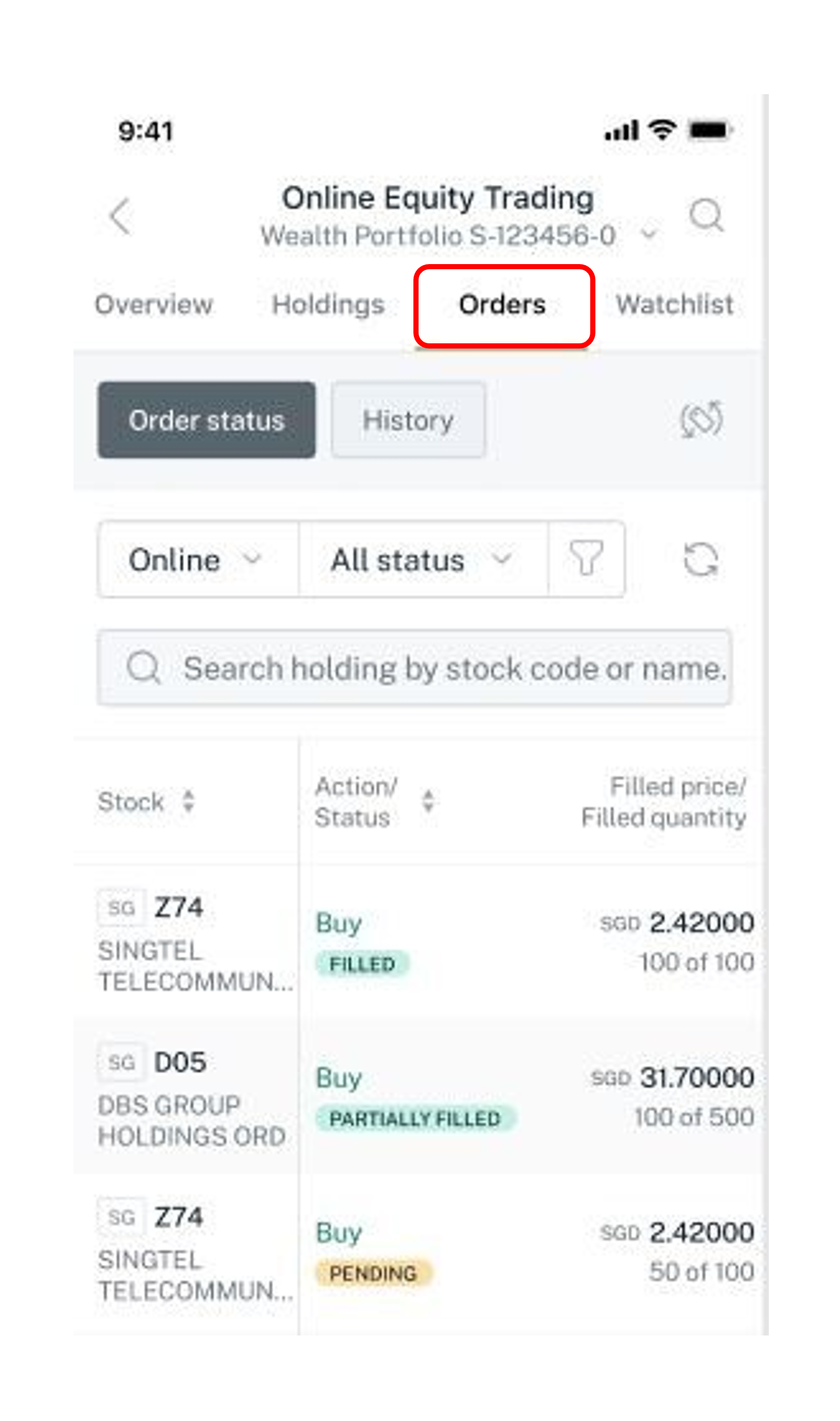Here is the cleaned-up and detailed caption for the given image:

---

The image is a screenshot of a smartphone displaying a trading application interface against a white background. At the top left corner, the status bar is visible in black, indicating the time as 9:41, with full reception, Wi-Fi signal, and battery life.

Below the status bar, the screen shows a black header titled "Online Equity Trading", with a grey subheading "Wealth Portfolio S-123456-0". Adjacent to this text is a grey magnifying glass icon. 

Underneath the header is a navigation bar containing four tabs: "Overview", "Holdings", "Orders" (highlighted with a red border), and "Watchlist". A thin grey line separates these tabs from the rest of the content.

The main content area is divided into two sections by background color and headings. The first section has a dark grey background with a white heading labeled "Order Status". The second section has a light grey background with a black heading labeled "History".

Further down, the background returns to white. Here, two tabs are present with white text on a black background, labeled "Order Status" and a grey rectangle with a grey magnifying glass icon and the text "Search holdings by stock holdings or name."

The detailed table in the main content displays several columns and rows. The first column, titled "Stock", lists various stocks with their codes and descriptions: "Z74, Singtel Telecommunications", "D05, DPS Group Holdings ORD", and repeats "Z74, Singtel Telecommunications".

The second column, "Action Status", shows various actions in color-coded statuses: "Buy, Filled" (in green), "Buy, Partially Filled" (in green), "Buy" (in green), and "Pending" (in yellow).

The final column, "Filled Price, Filled Quantity", lists numerical values: "2.420000", "31.700000", and "2.420000".

---

This caption provides a comprehensive description of the screenshot, making it easier for someone to visualize the layout and content without seeing the image.